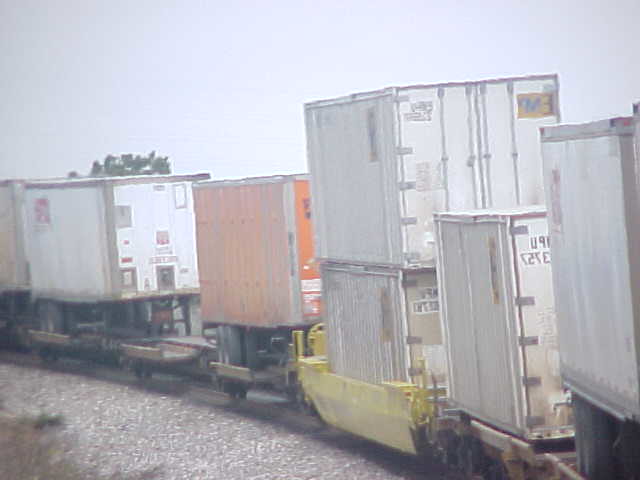This photograph is a grainy and overexposed snapshot that appears to be taken either through a window or in extremely bright lighting, resulting in muted and pale colors with minimal contrast. The image depicts a series of metal boxcar-like structures, likely train cars or containers, arranged one behind the other, extending from the right-hand side towards the middle left side of the photograph. These structures, primarily light gray or appearing white due to the overexposure, feature a central orange container overlaid with a silver-colored mesh.

The train seems to be positioned on a set of tracks that start in the lower right portion of the image and curve slightly as they extend off the left side. The tracks are bordered by gray gravel and some brush or grass in the bottom left corner. The cars, resembling flatbed train cars, carry various containers; one container car has two stacked containers, another has a single container, and additional cars carry containers mounted on wheels, ready to be transported by truck. The background features a blurry, washed-out sky and a solitary tree, adding to the overall muted and indistinct aesthetic of the scene.